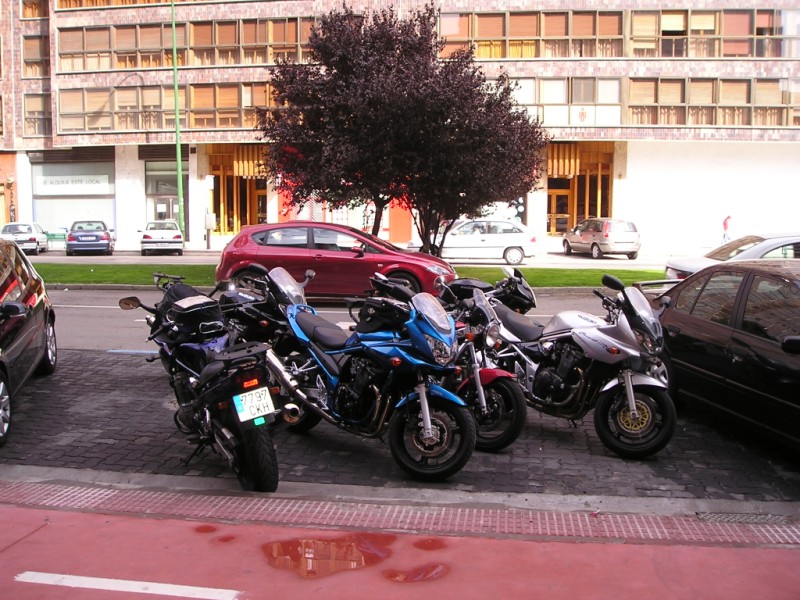The image is a color photograph of an urban street scene. At the bottom of the picture, there is a red concrete sidewalk with white stripes, possibly part of a bike lane, which also shows a small puddle. Adjacent to the sidewalk, there is a parking area paved with pavers, where a cluster of five to seven motorcycles in various colors (blue, red, silver, black) are parked together. Flanking the motorcycles are the edges of sedan cars on either side. 

Behind the parking area, there is a divided street with green grass and two small rounded trees on the median strip. The street features both pull-in parking spaces and cars parked side-by-side. A white vehicle is moving up the street, and a maroon-red Ford Fiesta type car is driving toward the right of the photograph, situated behind the back end of another small sedan.

In the background, a multi-story apartment or office building with a low, blocky structure is visible, though it's cropped off at the top. The building has an array of windows with shades, two wood-framed entrances, and striped awnings over the doors.